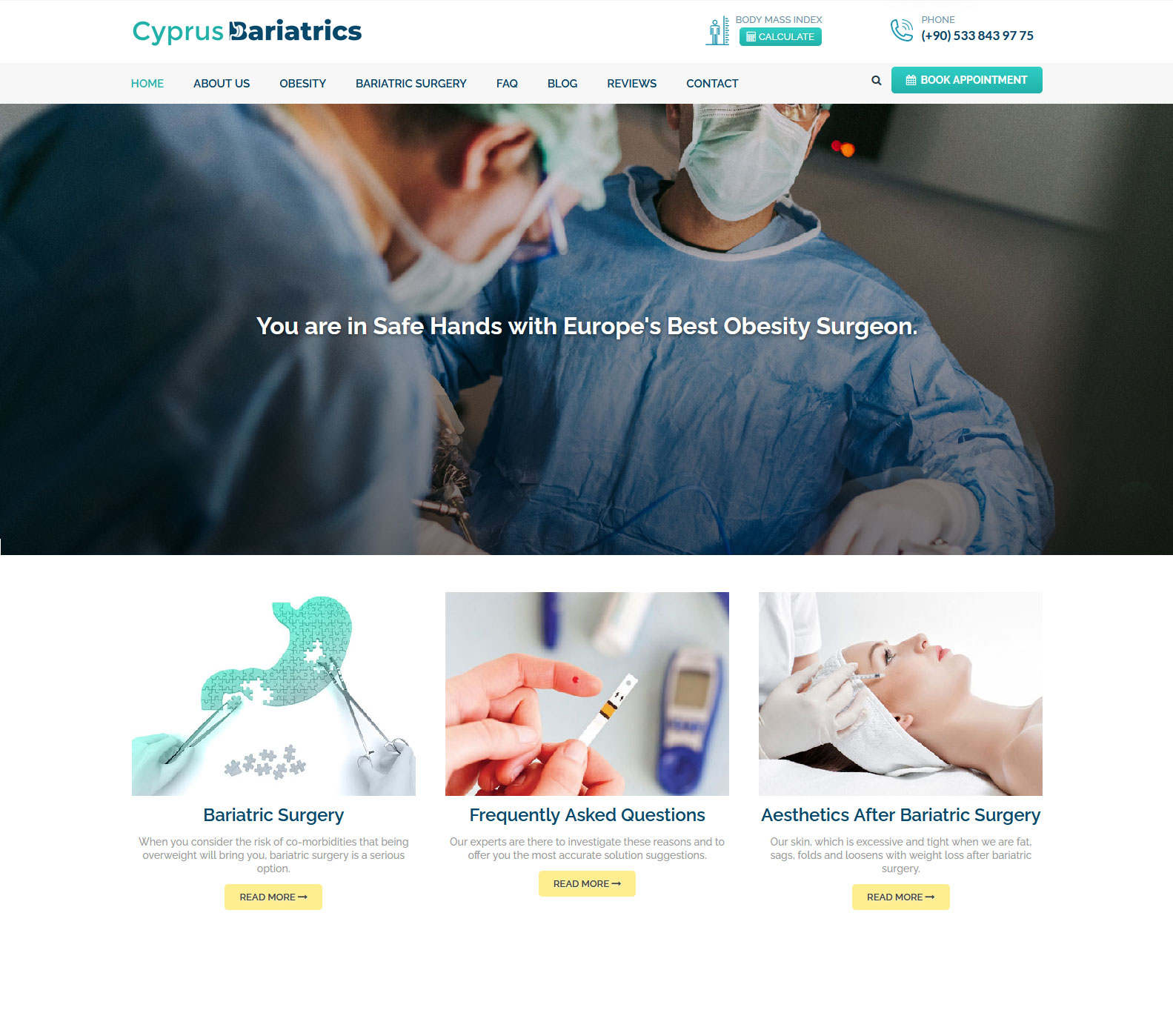This screenshot captures the homepage of a medical website dedicated to weight management and surgical solutions. At the very top, a white navigation bar features the site's logo on the left, labeled "Cypress Diuretics," rendered in a combination of teal and dark green. To the right, there's a Body Mass Index (BMI) calculator with a prominent green "Calculate" button, accompanied by a phone number for immediate contact.

Directly beneath this, a light gray horizontal bar hosts a series of navigation buttons: Home, About Us, Obesity, Bariatric Surgery, FAQ, Blog, Reviews, and Contact. Towards the far right of this bar, you'll notice a search function and a "Book Appointment" button, providing easy access for user actions.

The central portion of the screenshot is dominated by a large, high-definition image depicting a surgical scene where two surgeons face each other, emphasizing the expertise and professionalism of the medical team. The image is overlaid with bold white text that reads, "You are in safe hands with Europe's best obesity surgeon."

Below this compelling visual, the website features three columns, each presenting an article, presumably offering valuable insights and information related to obesity, medical procedures, and patient care. The layout is both visually appealing and intuitively designed to guide visitors through their health journey.